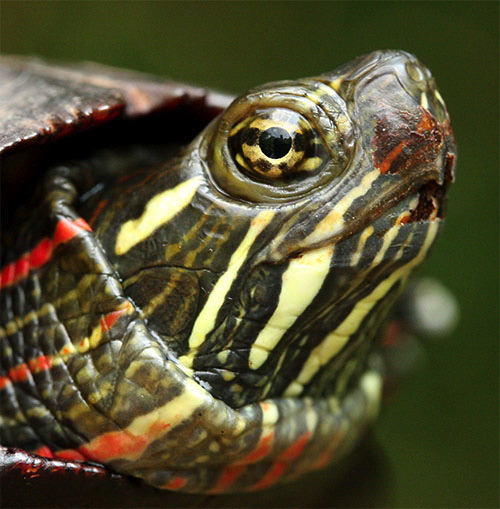This is a detailed square color photograph showing a close-up of the right side of a turtle's head, which is poking out from its shell. The image prominently features the turtle's head in the middle, slightly towards the bottom left corner, with the turtle looking towards the top right. The head displays a dark green hue with shiny, slick eyes that have a black pupil and yellow and black iris. Surrounding the turtle's eyes and extending down its neck are distinctive yellow and light yellow stripes, interspersed with a few red stripes that create an impression of red paint, making it seem like the turtle might be injured or bleeding. The turtle's skin, especially around the neck area, is also marked with reddish-brown elements. The background is characterized by a blurry green color, giving the setting a natural, wild appearance. Overall, despite the potentially alarming appearance, the turtle looks alert with wide-open eyes, suggesting it is aware of its surroundings.